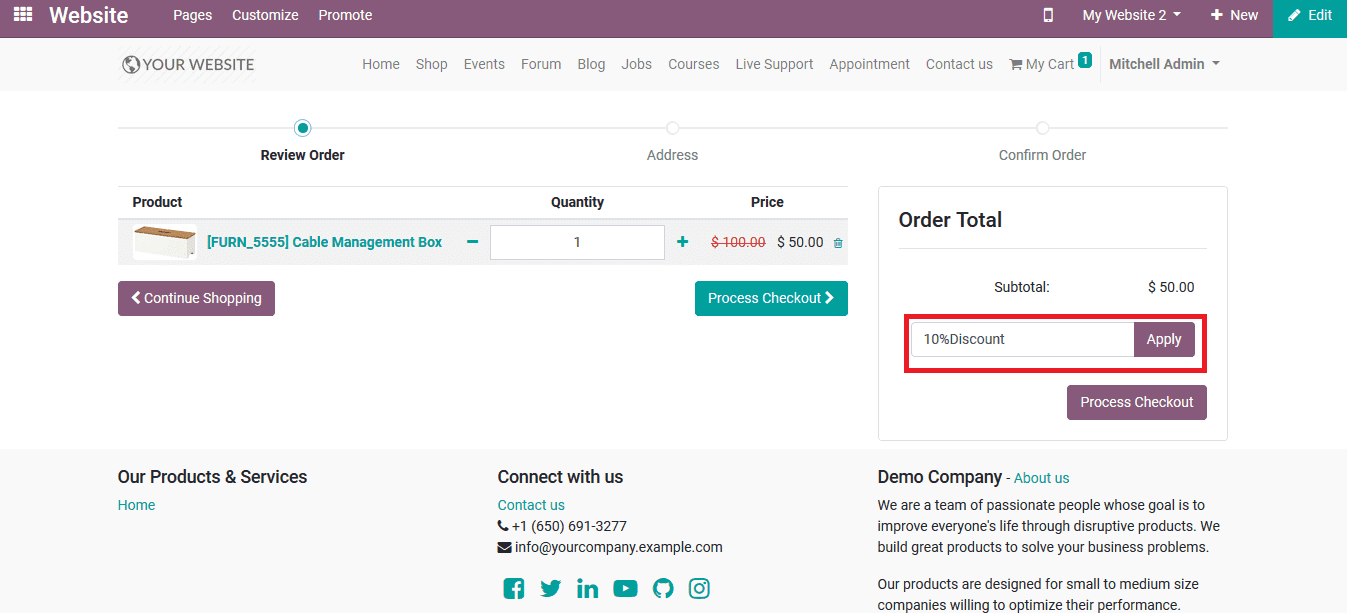**Detailed Description of a Demo Online Shopping Page:**

This image is a detailed, color screenshot of a demo online shopping website. The website design primarily features a clean white background with contrasting black text. At the top of the page, there is an aubergine-colored navigation bar that spans the width of the site. The right-hand side of this bar contains a green rectangular box with white text that reads: "Website," "Pages," "Customize," and "Promote." Adjacent to this text is a phone icon and the label "My Website" with a down arrow, indicating a dropdown menu. There are buttons for "New" and "Edit," with "Edit" highlighted in green.

On the left side of the page, the header "Your Website" is displayed next to a globe icon. Below this, there is a vertical navigation menu listing: "Home," "Shop," "Events," "Forum," "Blog," "Jobs," "Courses," "Live Support," "Appointment," "Contact Us," and "My Cart." The name "Mitchell Admin" is shown, suggesting the site administrator.

Underneath the navigation menu, there is a slider area featuring various tabs for reordering, addressing, and confirming orders. These include columns labeled "Product," "Quantity," and "Price." An example product listed is "FURN 5555," a cable management box, with an accompanying image depicting a white rectangular box with a brown top. The quantity listed is one. The original price of $100 is shown in red with a strikethrough, indicating a discount, and the current price is $50.

At the bottom of the product listing is a "Continue Shopping" button in aubergine on the left side with a back arrow, and a "Proceed to Checkout" button in green on the right side with a front arrow. 

Further down, there are sections labeled "Our Products and Services" and "Home." Contact details are provided, including a phone number, an email address, and social media icons at the bottom of the page. 

To the right, there is a rectangular section summing up the order's financial details, with "Order Total," "Subtotal: $50," a "10% Discount" section, and an "Apply" button in aubergine. This section is encased in a red rectangle. The "Process Checkout" button is also featured within an aubergine box. 

At the bottom, the site identifies as a "Demo Company," with an "About Us" section briefly stating: "We are a team of passionate people whose goal is to improve everybody's life through disruptive products. We build great products to solve your business problems. Our products are designed for small to medium-sized companies willing to optimize their performance." 

Overall, this image provides a comprehensive view of a demo online shopping page, highlighting its layout, features, and sample content.